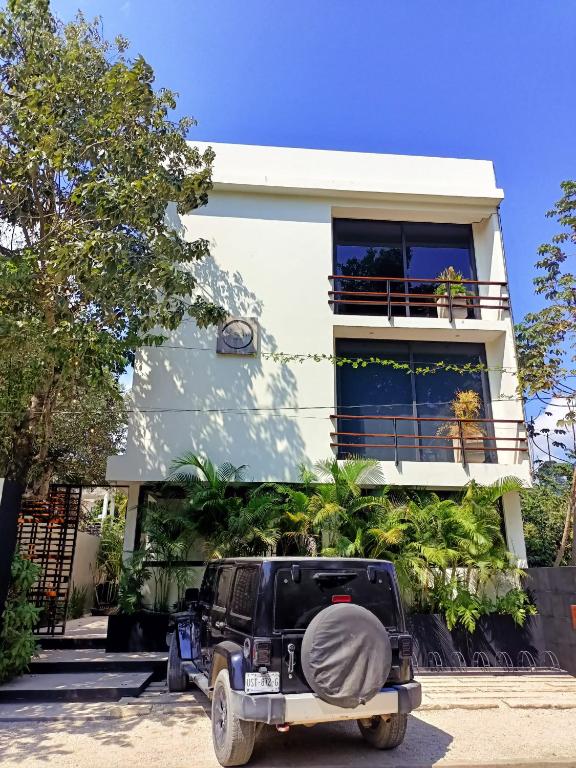This modern photograph showcases a pristine, two-story white house in a sunny area. The upper and lower stories each feature a balcony with neat metal railings, adorned with a potted plant on each. The house facade is plain and white, embodying a sleek, contemporary design. To the left of the house stands a large tree, only partially visible, casting shade over a wrought iron gate beneath. In front of the gate, steps lead up from the foreground where a blue and black Jeep with a gray tire cover is parked on a paved area. The lower part of the house is almost hidden behind tall palm trees that reach the height of the first floor. A bike rack with multiple slots is situated near the tree, adding to the functionality of the space. The scene is framed by a stunning, clear blue sky, adding to the vibrant, sunny ambiance of the location.